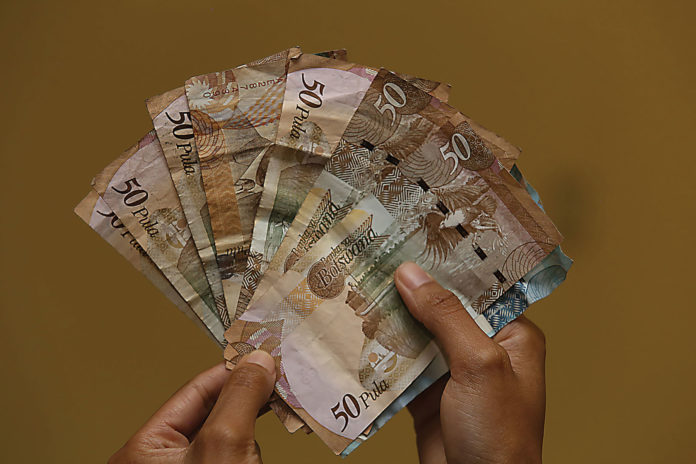The photograph captures a pair of dark-skinned hands holding a fan of eight identical banknotes against a brown painted wall. The image is horizontal, with the top and bottom sides twice as long as the left and right sides. The bills, labeled "Bank of Fibat Suana," each display the denomination "50" prominently in white on the top right corner and in black on the bottom left corner. The currency, tan and brown in color, is from Botswana and is marked "50 Pula" in brown lettering. Each bill depicts an eagle and a building in the background. The hands holding the money are positioned in the foreground, while only the brown wall is visible in the background.